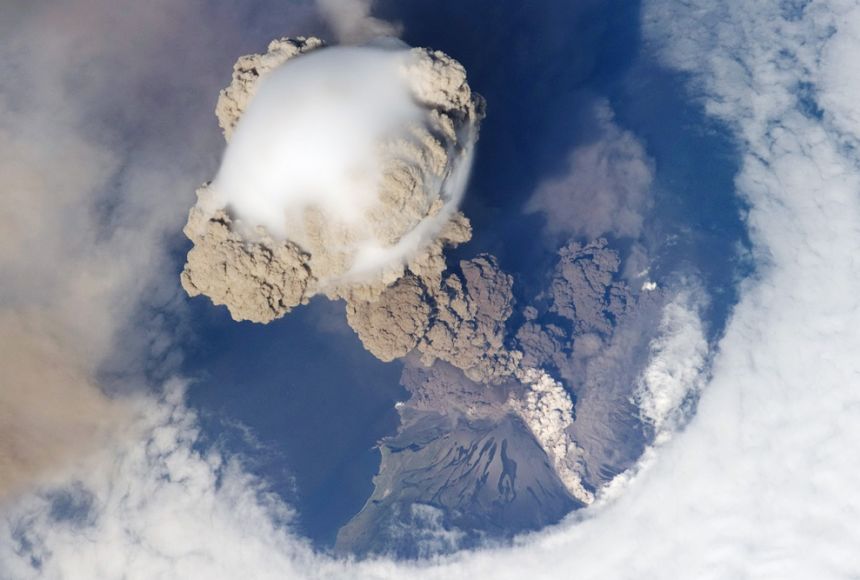This landscape photograph, taken from a high altitude, vividly captures a volcanic eruption. In the center of the image, a striking white cloud of smoke rises dramatically from the volcanic island below, even reaching and merging with an overhead cloud. The island, engulfed in the eruption's chaos, is surrounded by varying hues of blue ocean water that underscore its isolation. Beneath the island, clouds form a distinct U-shape, their texture becoming dirtier and darker towards the left side, likely due to accumulating volcanic ash and smoke. Smoke can be seen cascading down both the right and left sides of the island, possibly a result of the collapsing volcano and subsequent dust fallout. The top center of the image features a textured white circle with a grayish perimeter, further illustrating the dense smoke emanating from the eruption. The entire scene is enveloped in a mix of fog, white clouds, and multi-colored smoke, with shades transitioning from light at the top to darker grays and blacks towards the middle and bottom of the photograph, emphasizing the intensity and magnitude of the volcanic explosion.